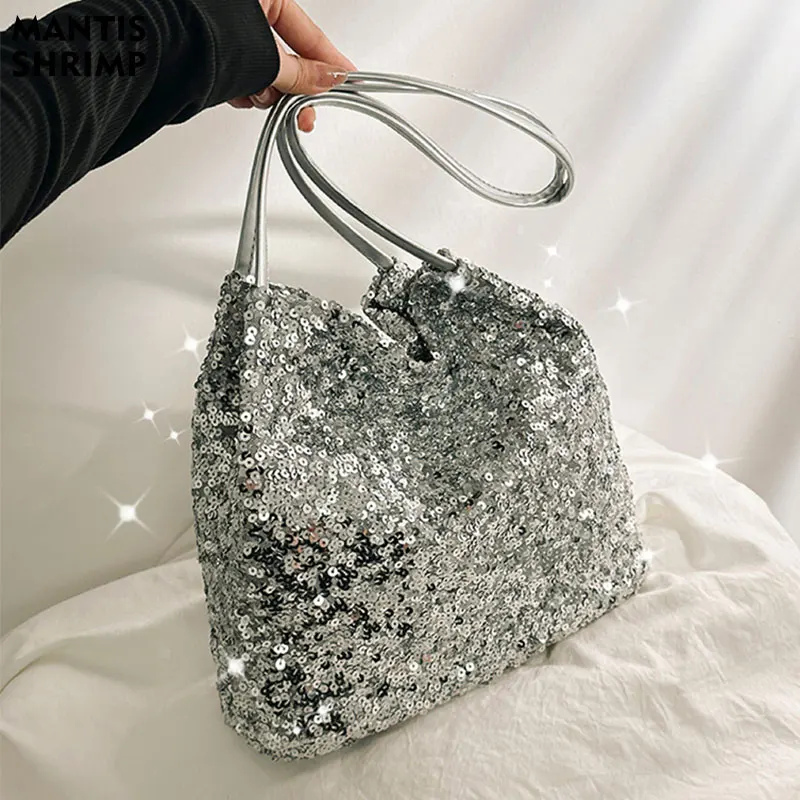In the photograph, a silver sequin purse, dazzling with numerous tightly packed shiny discs, is showcased against a white comforter and white sheet background, making its sparkle distinct. A woman, wearing a black ribbed long-sleeve shirt, is holding the purse by its silver double straps. Her outstretched hand, with nails painted in a nude color, delicately grasps the straps, highlighting the handbag's mid-size and elegant design. The white woman's careful presentation of the purse emphasizes its functionality as both a handbag and shoulder bag, with the straps looped to show their full length. The image captures the beauty of the purse, making it the focal point amidst the clean, contrasting backdrop.